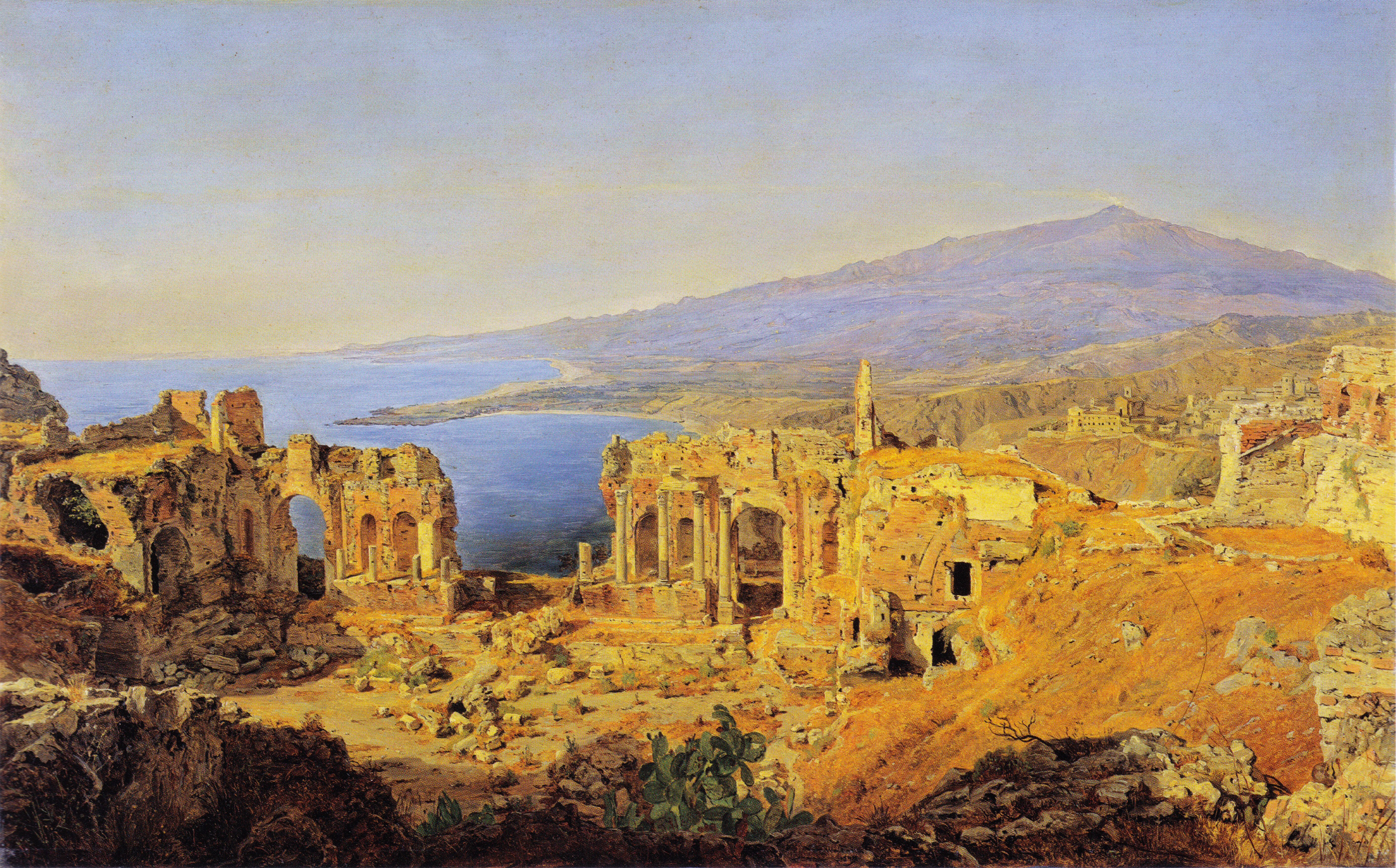The painting is a detailed landscape of ancient ruins, likely Greek, situated in a hilly or mountainous valley scene. Central to the image are tan, broken-down structures and numerous pillars, creating the impression of a once grand agora surrounded by jagged rocks in shades of grays and tans. The ruins sit on arid terrain bordered by steep cliffs devoid of vegetation. In the middle-right part of the image, there is a small body of water that occupies about 10 to 15 percent of the canvas, enhancing the depth of the scene. Adding to this sense is a distant mountain with a peak that rises almost pyramid-like from the landscape, accompanied by more rocky outcrops.

The background features a sweeping view towards the horizon, marked by a serene ocean on the left side of the image. The sky is a pale blue, transitioning into a sheet of nearly translucent clouds near the horizon. These delicate clouds barely mask the sky, allowing the warm sunlight to cast an almost golden hue over the ruins and barren earth. The overall color palette is warm, primarily consisting of light browns, tans, and muted greens, evoking a sense of antiquity and timelessness. Additionally, a small cat appears in the bottom center of the painting, subtly integrating life into this historic scene.